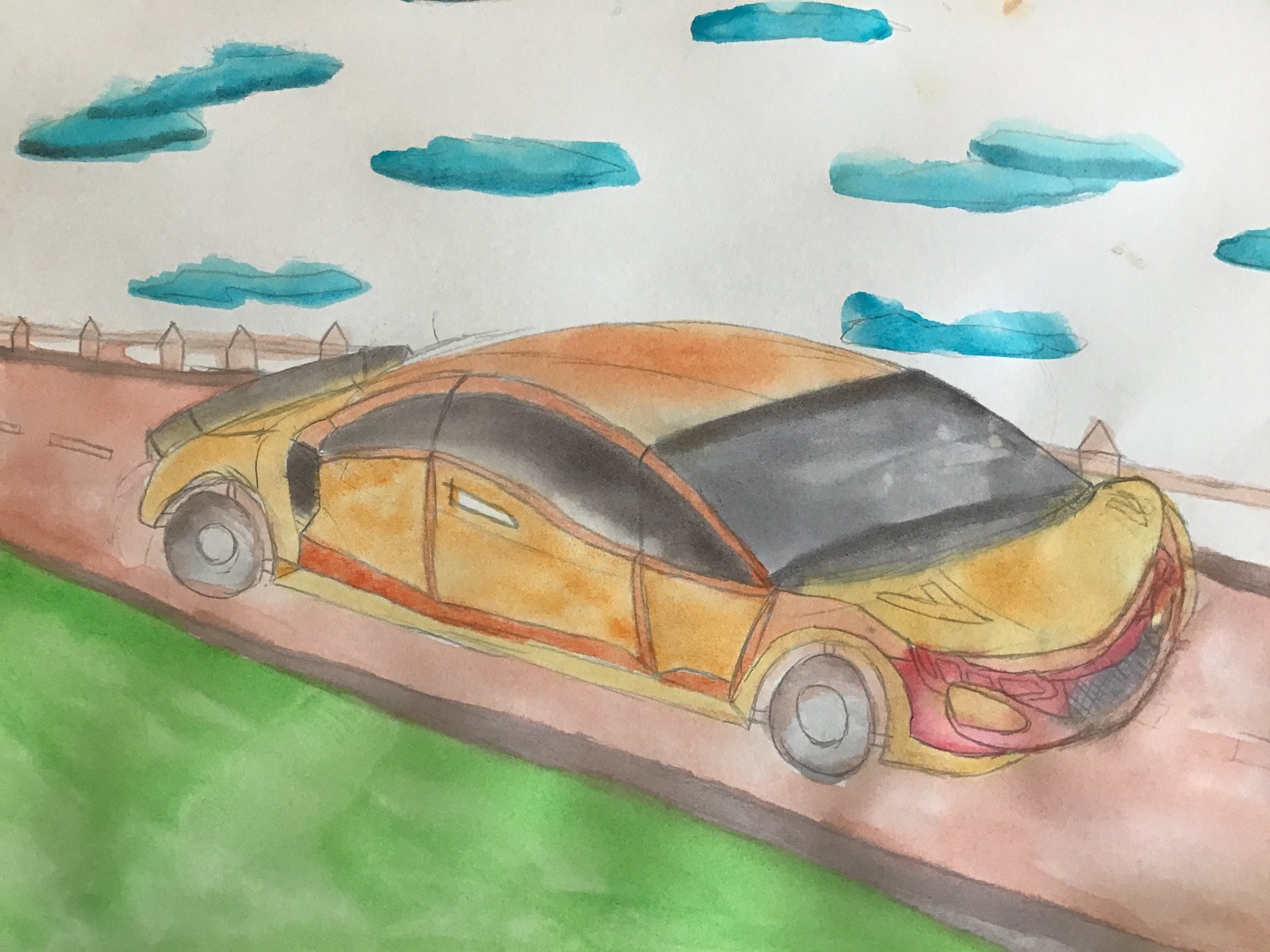This meticulously crafted artwork showcases a detailed depiction of a car set within a vividly painted outdoor scene. The initial sketch appears to have been executed in pencil, lending fine detail to the elements within the piece. Following this, watercolor paints have been meticulously applied to bring vibrant life to the scene. In the left corner, a solid expanse of green grass is prominently painted, providing a lush foreground. A road, rendered in a striking reddish tone with dark gray borders, cuts diagonally from the bottom right to the middle left of the composition, adding dynamic movement. Alongside the road, on the side farthest from the viewer, stands a rustic brown picket fence, adding an element of quaint charm. The sky, predominantly white, is streaked with delicate blue clouds, enhancing the scene's airy and serene atmosphere. Dominating the scene is a striking orange car, accented with a red bumper. The vehicle's wheels are colored in various shades of gray, while the windows are depicted in a stark black, offering a bold contrast. This artwork masterfully blends pencil sketch details with the rich hues of watercolor, creating a striking and harmonious visual narrative.